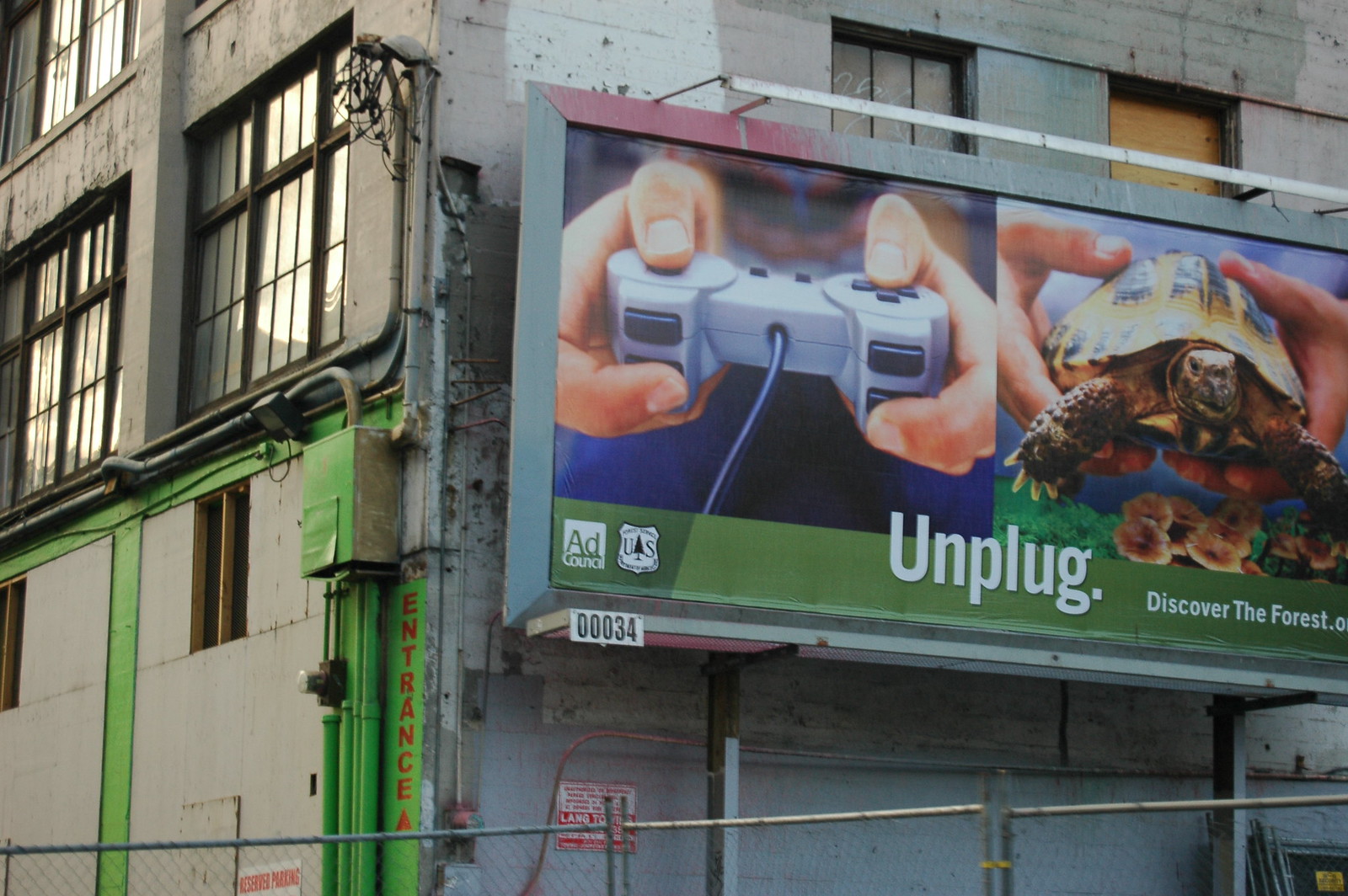This image captures the exterior corner of an industrial-looking building. The structure is predominantly cement, with a rough and unappealing look. The left side of the building is tan, while the adjoining side is gray. Tall, rectangular windows with black frames punctuate the walls. A striking lime green paint covers the corner where the two sides meet, prominently featuring the word "Entrance" written vertically in red.

Mounted on the gray section of the building is a sizable rectangular billboard with a metal frame. This billboard is partially visible, showing two distinct images. On the left, a close-up of hands gripping a wired, gray gaming remote control, likely a PS1 controller. Next to it, another set of hands holding a turtle with a yellow shell, against a background of coral. Below these images, the text "Unplug" is written in bold white letters. The bottom of the billboard displays a gray border with a touch of red at the top and another green section which partially shows the phrase "discover the forest," likely part of a larger call to action to visit nature. Additionally, a white rectangular sign with black numbers "00034" is visible at the bottom of the billboard. In front of the building is a small metal fence, indicating an area possibly used for parking.